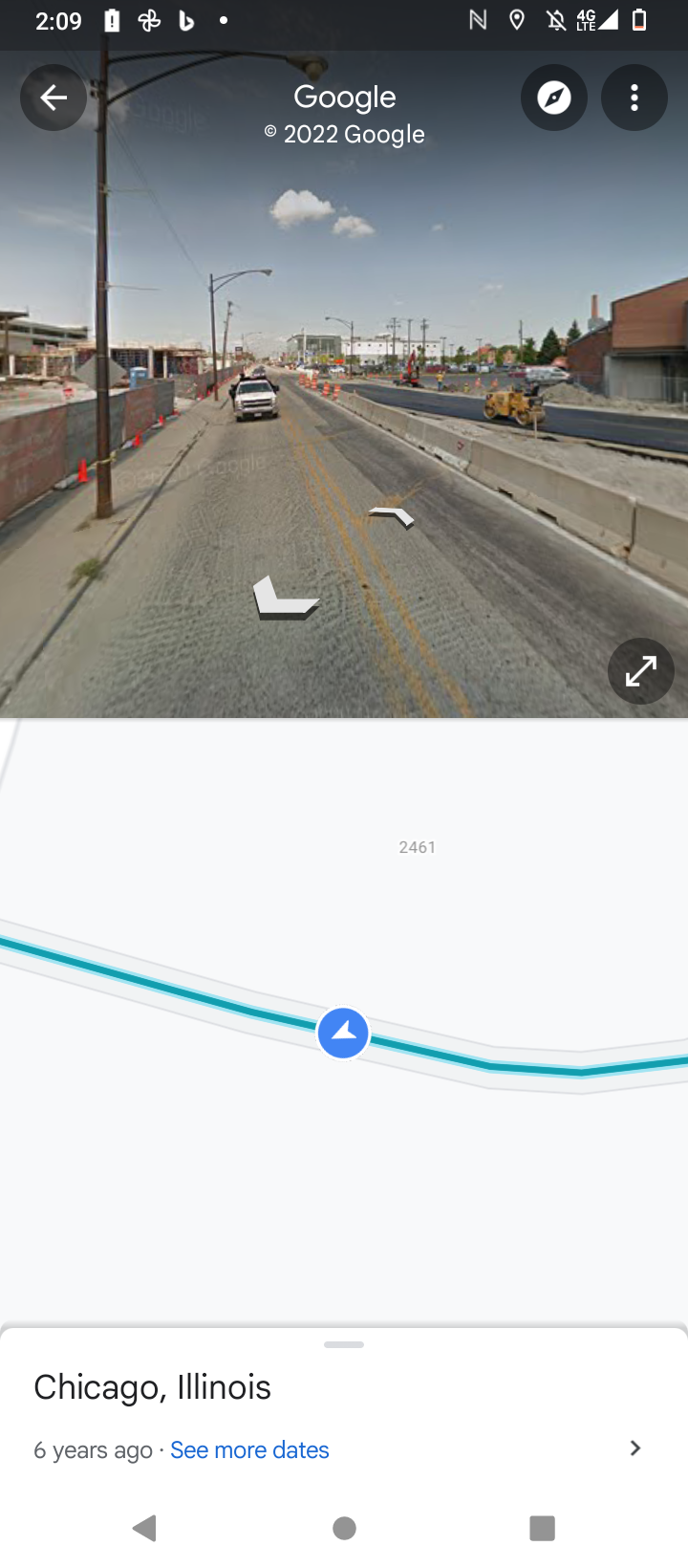This screenshot, captured on a mobile phone, prominently displays a Google Maps view of a city scene dated six years ago in Chicago, Illinois. At the top of the image, the phone’s status bar shows it is 2:09, the battery is nearly full, and several icons indicate active features such as 4G and location services. The screen captures a typical street view of a roadway bordered by buildings and light poles in the distance under a partly cloudy sky. The central focus of the image is a white truck driving towards the camera, positioned on the right side of a highway divided by a barrier, beyond which another lane of traffic can be seen. To the right of this barrier, a construction zone with orange cones and a brown building with a red roof is visible. Beneath the cityscape, there's a map interface with a prominent blue line and a blue circle featuring a white arrow, guiding navigation. Below this navigational symbol, the text reads “Chicago, Illinois, six years ago,” with a “see more dates” option underlined in blue.